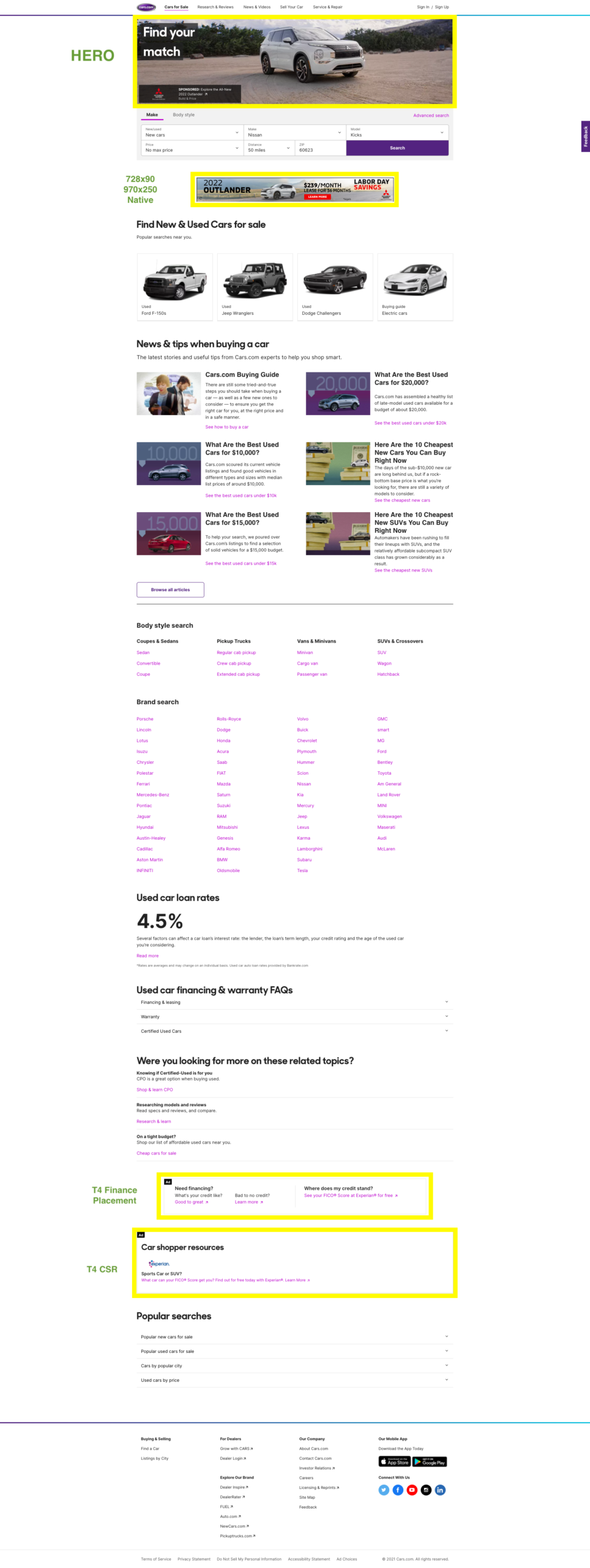The image captured on a cell phone screen portrays a person engaged in car shopping or attempting to sell a vehicle. At the top left corner of the screen is a picture of a white SUV accompanied by the text "Find your match" in white font. This section is highlighted with a yellow border, drawing attention to it. Below this, there are several information boxes intended for inputting details, followed by another highlighted section featuring the 2022 Outlander, which also appears to be a white SUV.

Further down the page, the screen displays a list under the heading "Find new and used cars for sale." This section showcases four vehicles: a white truck on the left, followed by a gray Jeep, a black sporty two-door car, and lastly, a white electric car. Each vehicle is visually distinct and separated into individual segments. At the bottom of the page, additional areas are similarly outlined in yellow, indicating sections of significance or input fields.